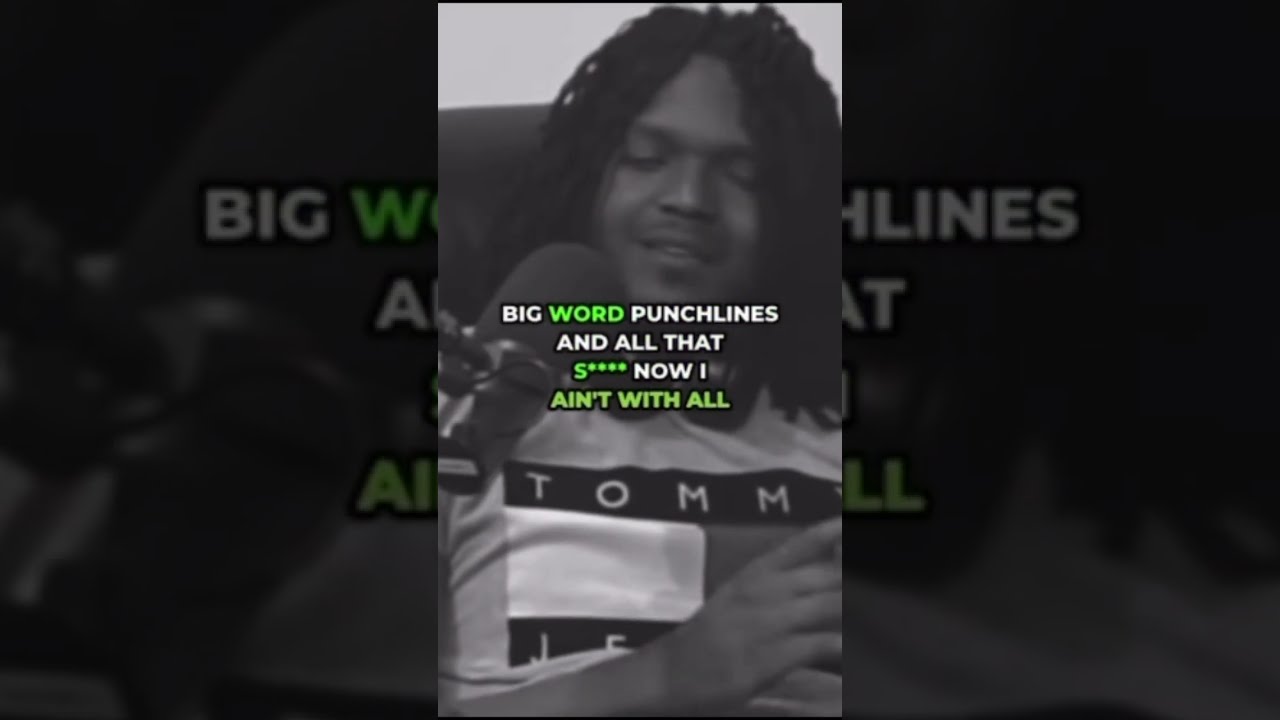The black-and-white image features a relaxed black male with dreadlocks, wearing a short-sleeved Tommy Hilfiger shirt, sitting in front of a pole-mounted microphone. He has a slight smile and closed or downcast eyes. The text overlaid in the center of the image reads "big word punchlines and all that. S*** now I ain't with all," with "big," "punchlines and all that," and "now I" in white and "word," "S***," and "ain't with all" in green. The same image is also used as a larger background, making it appear three times bigger than the main central image, continuously extending to the right and left. This setup gives the impression of a screenshot from an app like TikTok or Instagram.